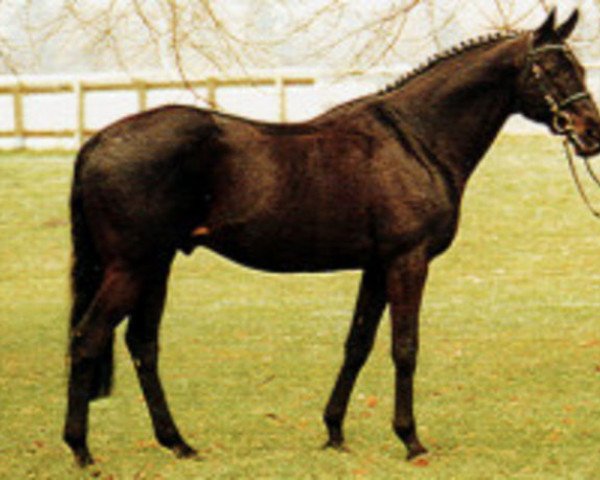In the photo, a medium to dark brown horse stands still in a lush, green grassy field. The horse, possibly male, is devoid of any saddle but wears a harness with reins that extend outside the frame, suggesting someone is holding them off-camera. Its mane has been intricately braided, adding to its groomed appearance. The horse faces to the right, revealing its long tail, although some details are slightly obscured due to the picture's slight blurriness. The background features a light-colored fence running along the edge of the property, with tree branches hanging down in front of and behind the fence, indicating a natural setting, possibly a ranch. Despite some dark and light shading variations on its coat, likely influenced by lighting, the horse's overall color remains consistently deep brown.